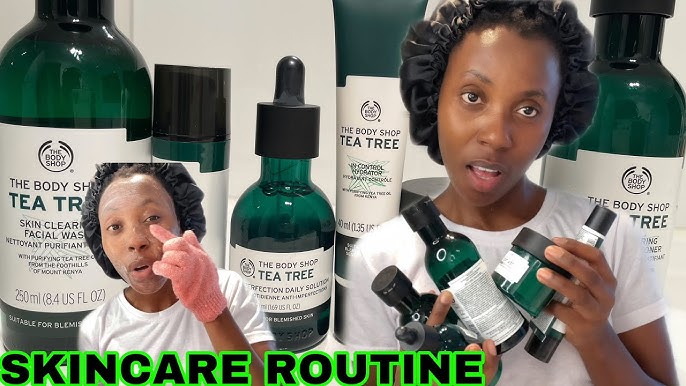This composite YouTube thumbnail for a skincare routine video features a dark brown-skinned African American woman wearing a hairnet and a bonnet to keep her hair secured. The woman is seen holding a selection of green-colored bottles from The Body Shop’s Tea Tree range, which include products such as Skin Cleanser, Facial Wash, Imperfection Daily Solution, and In Control Hydrator. The thumbnail is divided into two sections: on the left, the woman is shown washing her face using one of the Tea Tree products with a pink glove, while on the right, she holds up five different Tea Tree products. The bottom left corner of the thumbnail prominently features the text "skin care routine." The images are overlaid on one another, emphasizing the various steps and products involved in her skincare routine.